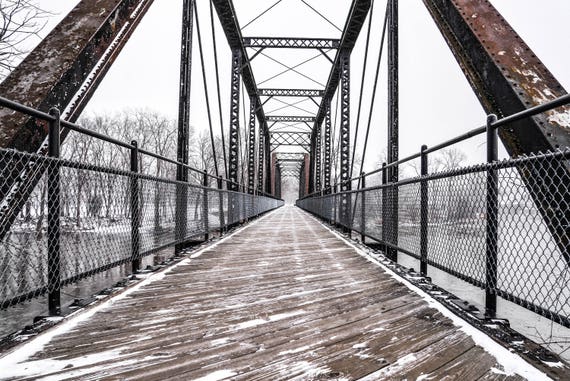The image depicts a long, old bridge stretching across a body of water on a cold winter's day. The bridge is primarily composed of wooden planks, with intricate wooden diagonal pieces creating its structure, all dusted with a light covering of snow. The supports of the bridge are made of rusted metal beams and steel cables that run from the top to the bottom, providing stability. On either side of the bridge, there are chain link fences and metal gates that add a sense of enclosure. Overhead, large metal beams intersect and connect, adding to the aged and industrial aesthetic of the bridge. The view looks across the length of the bridge to the opposite bank, where snow-covered ground and barren trees devoid of leaves are visible, reinforcing the winter setting. The sky above is uniformly gray, suggesting a heavy overcast with significant moisture in the air, contributing to the overall cold and somber atmosphere of the scene.